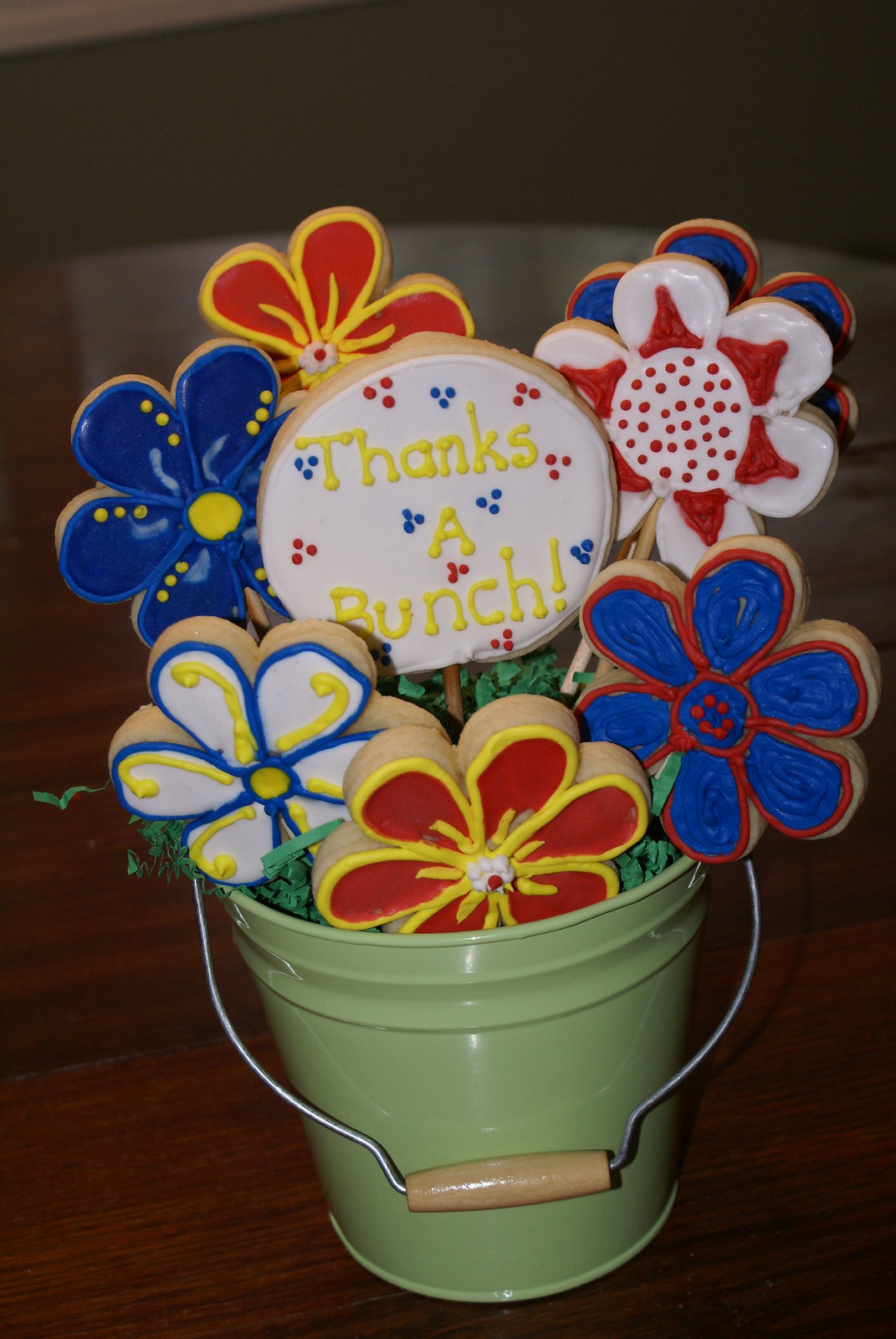This indoor image features a charming cookie arrangement set on a wooden surface that could either be a hardwood floor or a wooden table. At the center of the image is a small green bucket with a silver handle, equipped with a wooden dowel for comfortable holding. The bucket is filled with decorative Easter grass, which supports seven vividly colored sugar cookies shaped like daisies, each on a dowel rod. The cookies come in an array of colors, including red, yellow, blue, and white, with each flower meticulously frosted. The focal point of the arrangement is a round sugar cookie in the center that bears the message "thanks a bunch" in yellow icing on a white background. The photo, likely taken with a flash, captures the delightful details of the setting, making each element distinctly visible despite the otherwise dimly lit indoor environment.